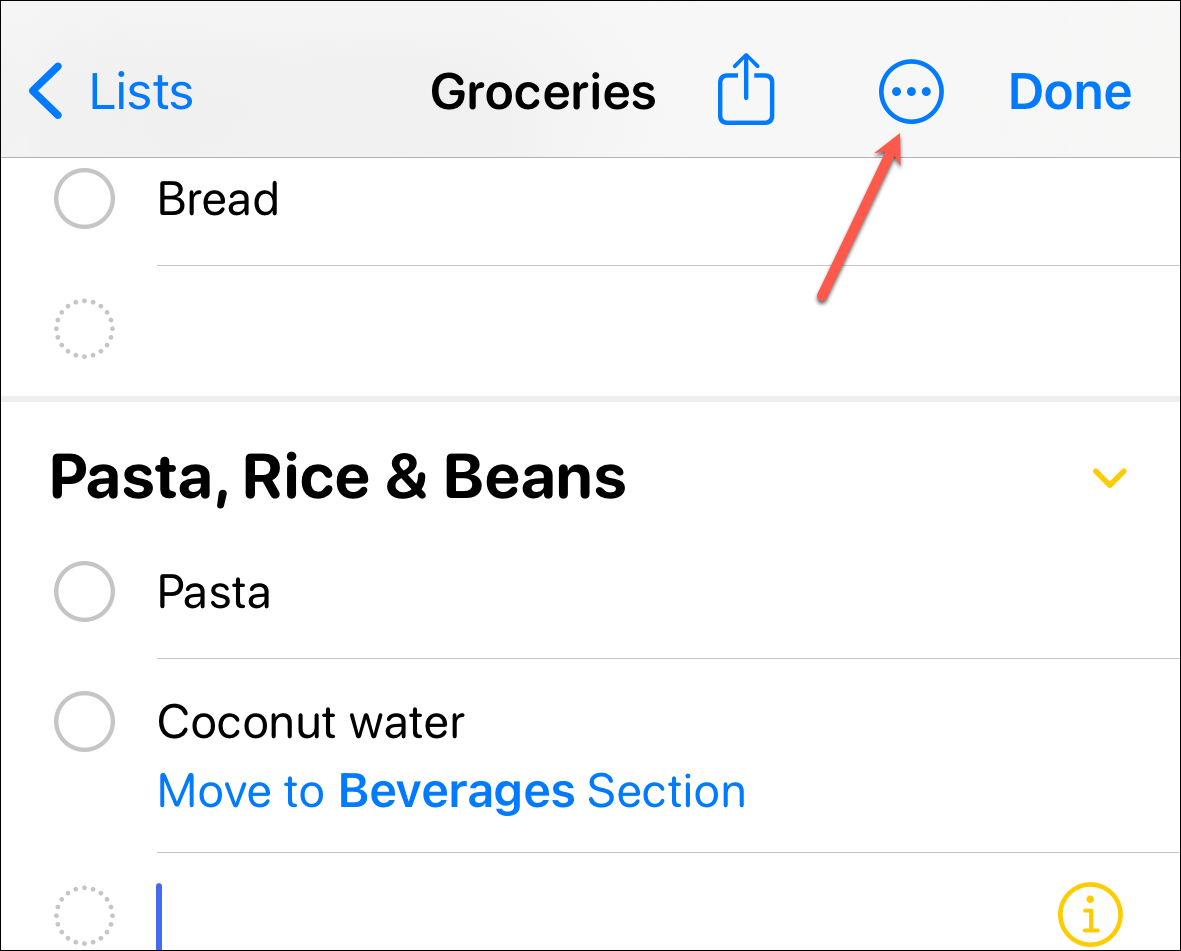This screenshot, taken from a tablet or smartphone, showcases a section of a webpage dedicated to creating and organizing a grocery list. At the top of the screen, a dark gray bezel frames the interface. On the left-hand side, a dark blue arrow accompanied by dark blue text reads "List." Centrally, the header "Groceries" is displayed in black text. Below it, a square icon featuring a blue arrow pointing upwards signifies an upload function. Adjacent to this icon, a red arrow directs attention to a blue outline circle containing three blue ellipses, likely representing settings or editing options. On the far right, the word "Done" is prominently displayed in bold blue text.

On the left-hand side, a series of circles represent checklist items. The first circle is labeled "Bread." The next circle, which is dotted, currently has no associated item. The subsequent section lists "Pasta, Rice, and Beans" in bold black text. To the far right of this section, an orange arrow points downward.

Further down, another bullet point marked "Pasta" appears in black, followed by another entry reading "Coconut Water." Below this, "Move to" is written in blue text, followed by "Beverages" in bold blue text, indicating a category or section move function, and then "Section" in regular blue text.

Another dotted circle with a cursor-like object glowing blue appears on the left-hand side, indicating an active selection. On the right of this is an orange circle with an orange outline, a white interior, and an orange icon resembling an eye, likely representing a visibility or viewing option.